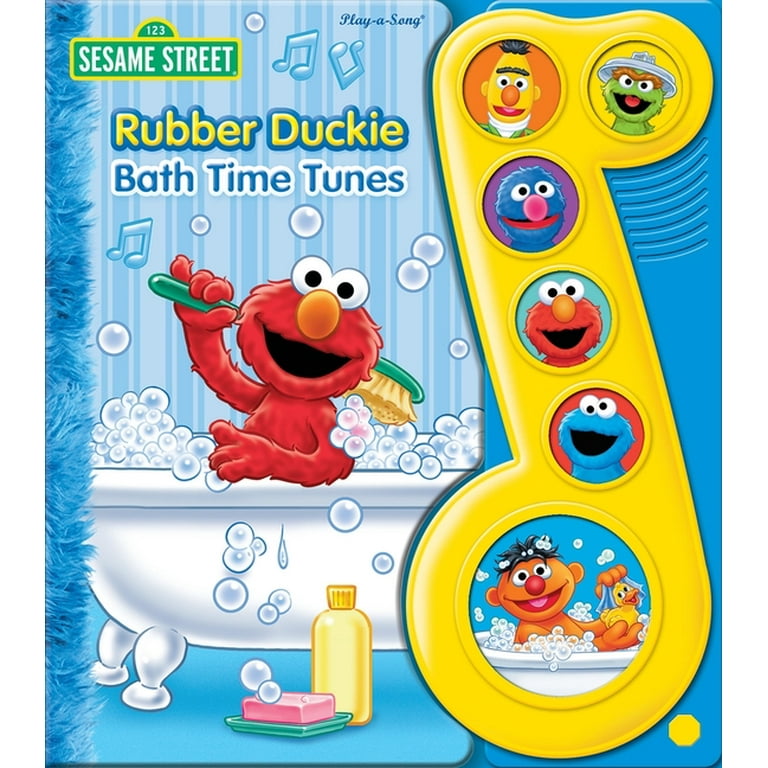This image shows a Sesame Street-themed children's play-along musical book titled "Rubber Ducky Bathtime Tunes." The book has a blue cover with a white claw-foot bathtub filled with bubbles and Elmo, who is depicted scrubbing his back with a green brush. The Sesame Street logo is positioned in the top left corner, followed by the title "Rubber Ducky" in yellow text and "Bath Time Tunes" in blue text below it. To the right of the cover is a yellow, plastic musical note with six distinct buttons, each representing different Sesame Street characters: Ernie, Cookie Monster, Elmo, Grover, Bert, and Oscar the Grouch. Each character button is in a different color and pressing them produces a sound. Adding to the playful bath scene, a yellow bottle of shampoo and a pink bar of soap are placed on the floor next to the tub. Elmo appears to be singing, with little musical notes coming from his mouth, enhancing the interactive fun for children. The book is designed with a sturdy cardboard material for durability.